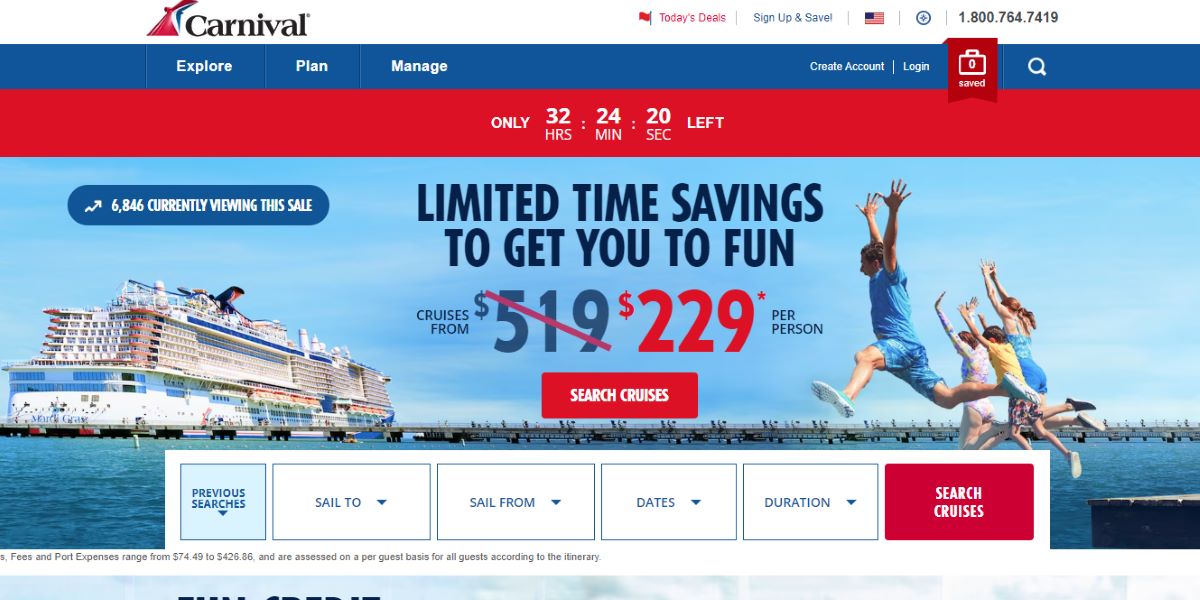This image is an advertisement for Carnival Cruise Lines, featuring a detailed layout with various elements designed to attract potential customers. At the very top of the ad, the name "Carnival" is prominently displayed in black text, accompanied by their red, white, and blue logo to the left. Below this header, there's a dark blue horizontal rectangular menu bar with white text categories including: "Explore," "Plan," "Manage," "Create Account," and "Log In." To the right of these categories, a red square with a white camera icon and the word "Saved" in white text is visible.

Further down, a red horizontal rectangle spans the width of the screen, highlighting a countdown with white text that reads, "Only 32 hours, 24 minutes, 20 seconds left." Below this, the main image captures a picturesque scene: a large Carnival cruise ship docked on the left, with a backdrop of a clear blue sky and tranquil blue water. A long dock extends towards the boat, creating a scenic view. To the right, there are four individuals— a man, a woman, and two children— joyfully jumping in the air.

In the foreground of the image, black text boldly declares, "Limited Time Savings to Get You to Fun." Just below, discounted pricing is displayed with "Cruises from 519," where "519" is crossed out with a red diagonal line, and the new price "$229 per person" is shown in red text.

Below these text blocks is a red rectangle with "Search Cruises" in white text. Following this, there are clickable options for customizing searches, including previous searches, destinations ("sail to" and "sail from"), dates, and durations. The "Search Cruises" option is highlighted in red with white text, while "Previous Searches" appears in a light blue box.

Displayed prominently at the bottom of the advertisement is a dark blue oval banner with the text "6,846 currently viewing this sale" in white, adding a sense of urgency and popularity to the offer.